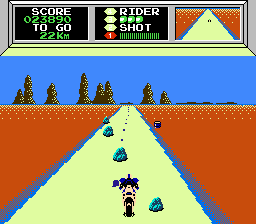This image showcases an action-packed moment of a video game in progress. At the top of the screen, there are three distinct panels. The leftmost panel, with a white overlay, displays the player's current score, "023890," and the distance remaining in the game, "222 km," also in white text. The central panel, set against a black background, features the word "Rider" in white, followed by three green dots, and the word "Shot" in white text. Below this, there is a red background displaying the number "1," along with several bars indicating progress or health.

The third panel to the right depicts a detailed, game-map-like display. A white triangle outlined in blue stretches out over a burnt orange landscape, representing a long road. Two tiny figures traverse this path, hinting at player or NPC (non-player character) movements.

Dominating the lower part of the screen is a large portion of this road, also outlined in blue, with one of the players centrally positioned on it. There are some blue objects on the road, though their specific purpose remains unclear. The entirety of the road is flanked by burnt orange-colored terrain. In the background, a vivid blue sky stretches out with several large trees dotting the horizon, adding depth and natural beauty to the game's immersive environment.